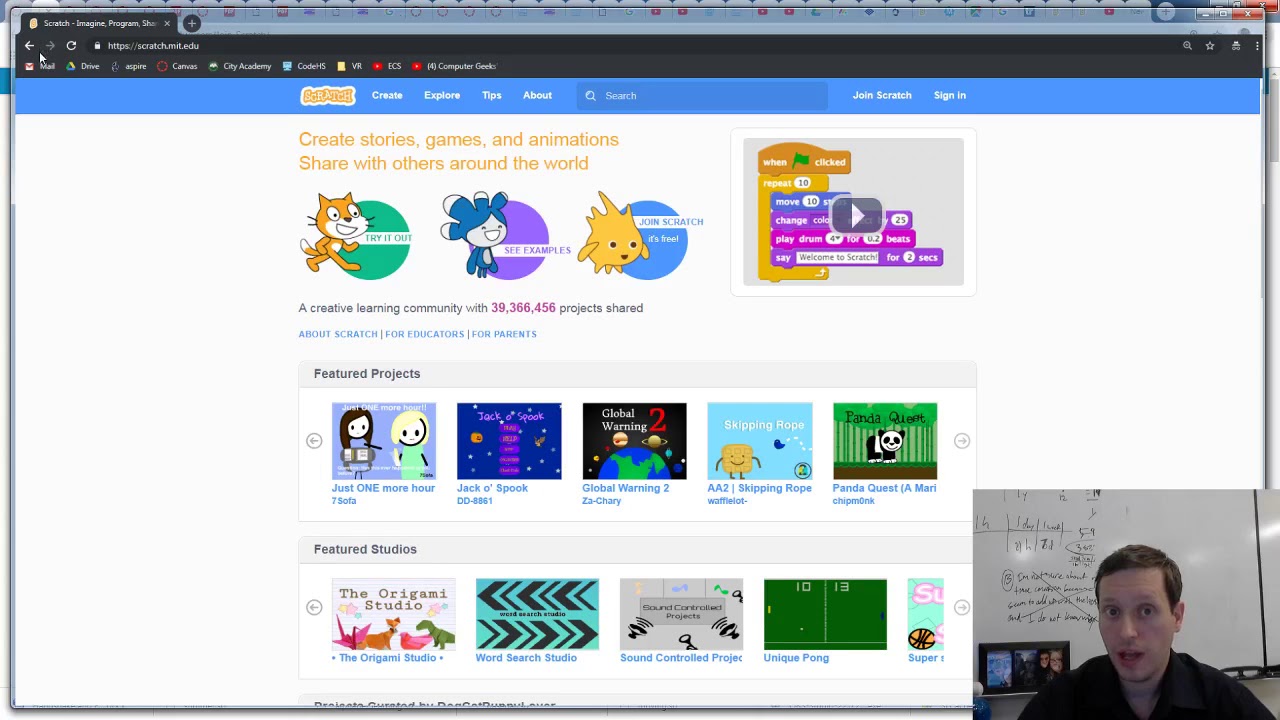The image appears to be a screenshot of a computer screen displaying the Scratch website, a platform for creating and sharing stories, games, and animations. At the very top, there's a black border indicating the browser window, with the Scratch URL visible. Below this, a blue navigation bar provides several options including 'Create,' 'Explore,' 'Tips,' 'About,' a search bar, and buttons for 'Join Scratch' and 'Sign In.'

The main section of the webpage has a white background with a prominent message inviting users to "Create stories, games, and animations. Share with others around the world." Below this text are three circular buttons, each accompanied by a unique character. The first button, labeled 'Try it out,' features a tiger next to a green circle. The second button, 'See examples,' is next to a character resembling a girl with blue and white hair. The third button says 'Join Scratch, it's free,' accompanied by a yellow creature.

In the center of the screen, there's a square with a play button, presumably a video or interactive tutorial. Towards the bottom of the page, two sections titled 'Featured Projects' and 'Featured Studios' display lists of highlighted projects with thumbnail images.

In the bottom right-hand corner, a pop-up appears to show a person in front of a whiteboard, seemingly conducting a lesson. The overall design is clean and educational, aimed at encouraging creativity and learning.